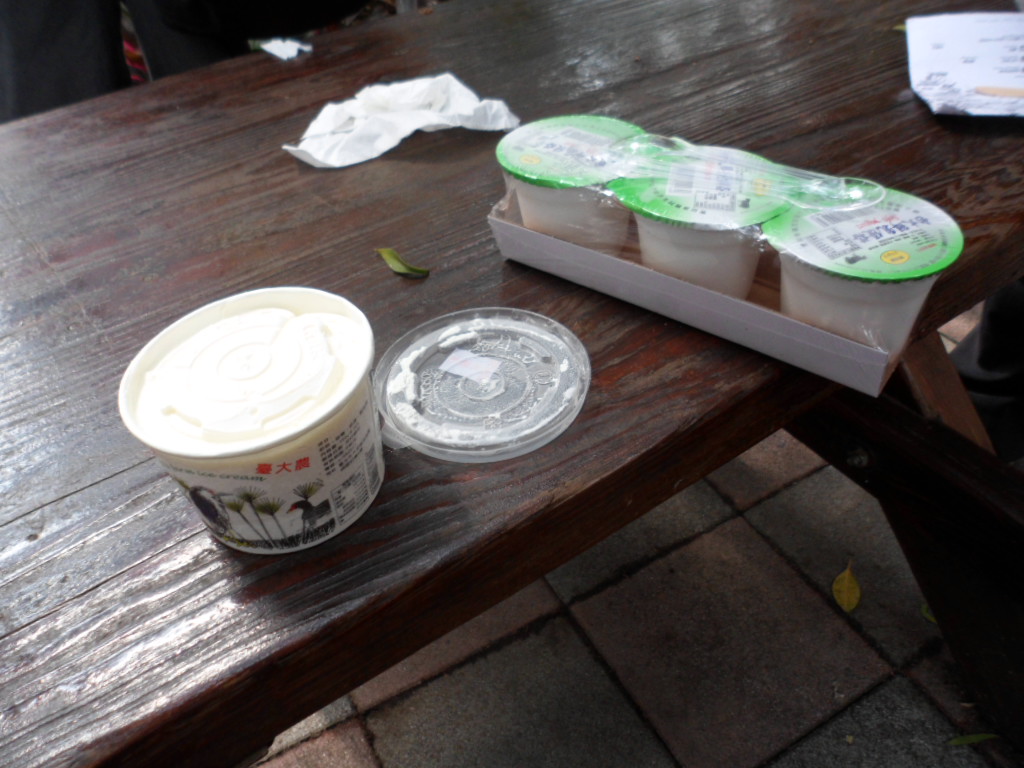The image depicts a close-up view of a dark brown picnic table with a tiled floor beneath. Positioned prominently on the table are various containers of a white substance, possibly ice cream, pudding, or yogurt, each adorned with distinct labeling and packaging.

To the left, there is a larger, open container with an unattached, clear plastic lid placed upside down next to it. This container features intricate designs, including black images that may depict birds or trees, complemented by red lettering in an Eastern Asian language, likely Chinese or Japanese. The contents inside appear untouched.

Adjacent to the larger container, there is a set of three smaller containers arranged in a line. These have green and white plastic lids with colorful designs and text, also in Eastern Asian script. They are secured together atop a white cardboard base and are accompanied by plastic spoons.

Central to the display, a used tissue and a piece of paper with indiscernible text are scattered casually, emphasizing the informal atmosphere of the setting. The overall scene suggests a dessert arrangement, perhaps left over from a recent meal or picnic.